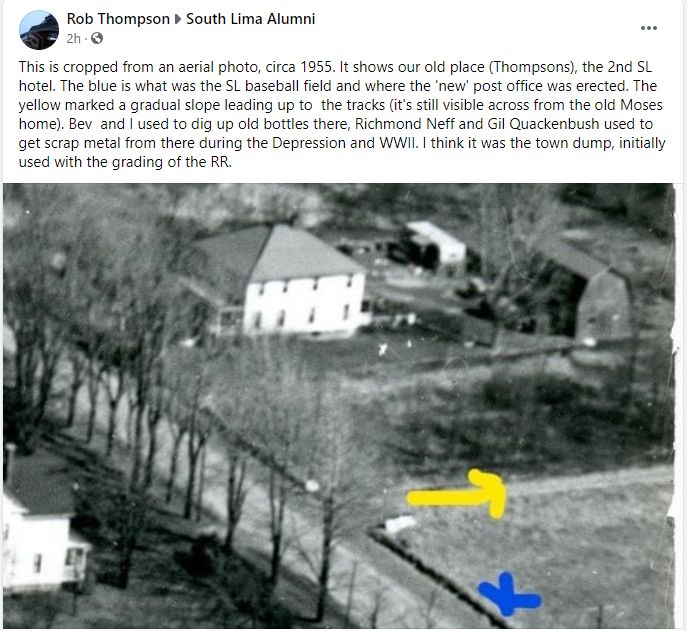This is a detailed description of a screenshot from a social media post, likely Facebook, authored by Robert Thompson. The post features an aerial black and white photo from circa 1955, depicting a farm area with a few buildings and a road. The text, displayed at the top of the screenshot, explains that the photo is of "our old place," including Thompson's, the location of the second SL hotel. It highlights key details with colored markers: a blue 'X' indicating the old SL baseball field and the site of a new post office, and a yellow arrow marking a gradual slope leading up to the tracks, a feature still visible across from the old Moses home. Robert reminisces about digging up old bottles with Bev in this area, and mentions Richmond Neff and Gil Quackenbush collecting scrap metal there during the WWII depression. The visual elements in the screenshot include different shades of gray in the photo and colored markers in blue and yellow on the image. The post details are surrounded by typical Facebook interface elements: Robert Thompson’s name, a small profile picture, a globe icon, and three dots for additional options.